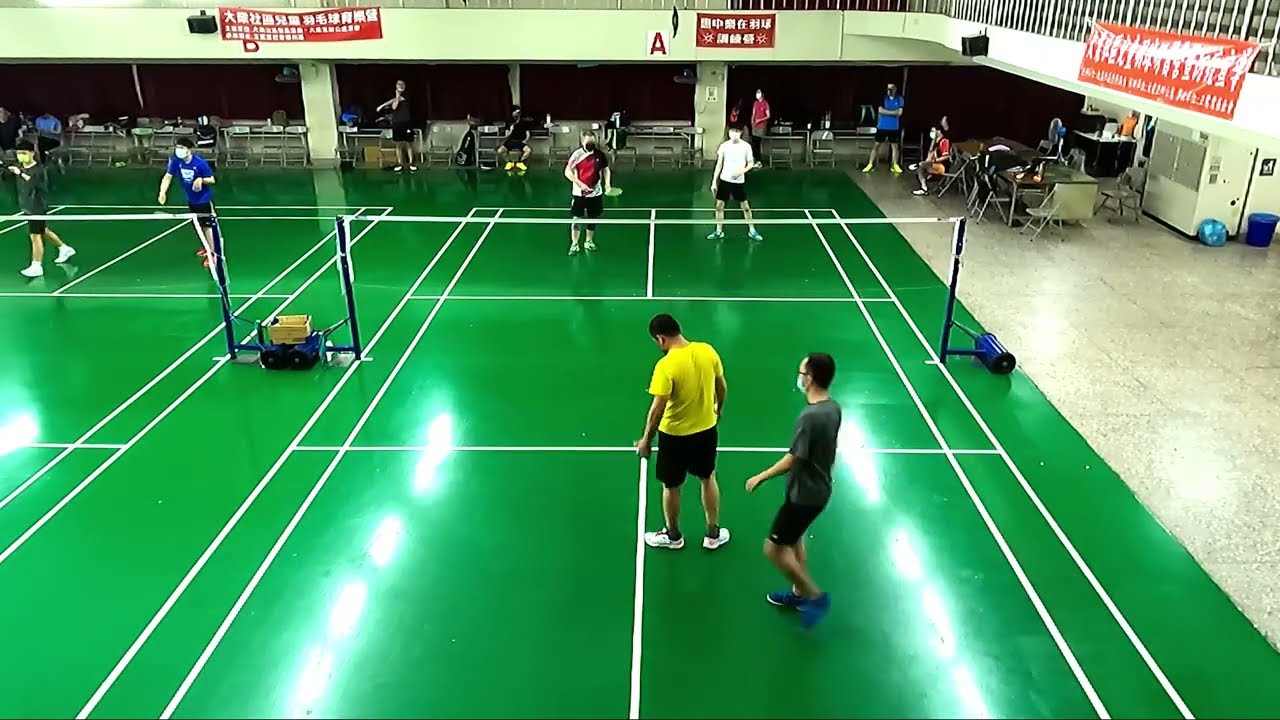This detailed photograph captures an indoor badminton court from an elevated perspective, revealing two adjacent courts, each with a green surface marked by white lines delineating various play areas. The courts are divided by white nets supported by blue poles. On the right side, beyond the courts, the floor transitions to tan and gray tile. The second story is visible at the top right, distinguished by a white painted railing and adorned with three red banners featuring white text.

Each court is occupied by two pairs of players actively engaged in a game. The players nearest to the camera have their backs turned; the individual on the left wears a yellow t-shirt, while the one on the right is in gray. Facing them on the opposite side of the net, one player sports a red and black shirt, and the other is clad in white. The adjacent court to the left is also in play, with another team competing.

In the background, along the green walls decorated with foreign-language posters, benches and seating arrangements are visible, populated by spectators who are either seated or milling about. This lively scene underscores the communal and recreational atmosphere of the indoor badminton facility.